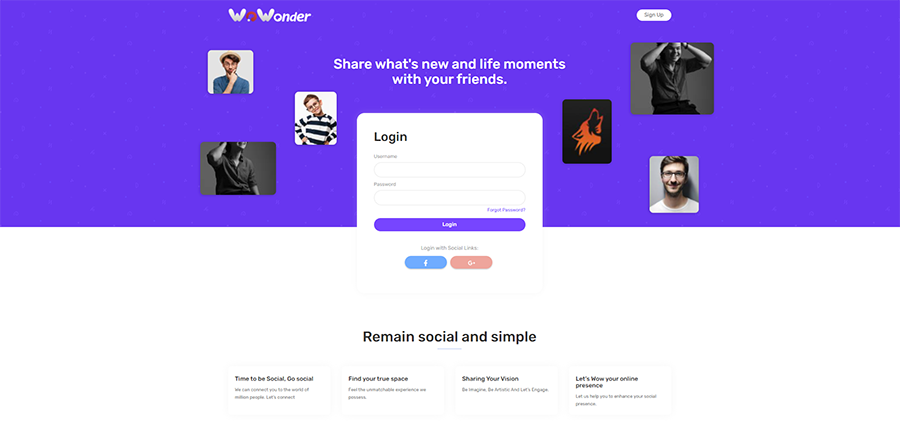This is a screenshot of a login page for a social media platform, possibly named "WOWonder" or "W-O-Wonder." The login area is set against a bold purple background. In the upper left corner of this area, the platform's name is prominently displayed, spelled out as "W-O-W-O-N-D-E-R" with the first "O" stylized as a red circle featuring a small dot in the bottom left.

At the center of the purple rectangle, there is a montage of images depicting five men who appear to be in their late 20s to early 30s. Alongside these images, there is a logo featuring a wolf howling at the sky. The text within this graphic encourages users to "Share what's new in life moments with your friends."

The login form is situated below this motivational prompt, containing blank fields for a username and password. The login button is also purple, maintaining the color scheme of the page. Beneath the login button, there are quick links to log in via Facebook and Google Plus.

A white banner stretches across the bottom of the page, bearing the slogan "Remain social and simple." Below this banner, there are additional links that likely lead to articles or other sections within the website.